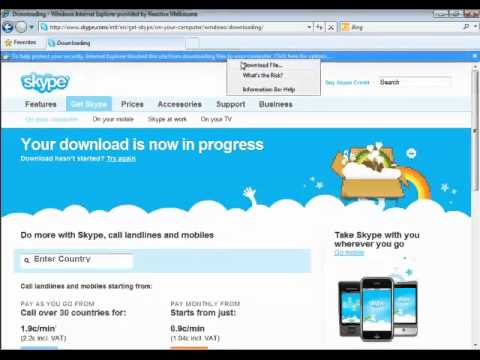The screenshot appears to be from an older version of the Skype website, focused on the "Get Skype" section. At the top, there is a traditional browser header showing the web address, which is partially visible as Skype. Below the header, the prominent Skype logo is displayed. The navigation bar includes tabs for Features, Get Skype, Prices, Accessories, Support, and Businesses, with the "Get Skype" tab currently highlighted in blue.

The central area of the page features a large blue notification that states, "Your download is now in progress." Below it, there is a message indicating, "If your download hasn't started, try again," with a background resembling a comic book style cloud image. Within this, there are colorful graphics including a cloud and potentially a rainbow or box element, likely indicating the download status visually.

Further down, a section titled "Do more with Skype" is visible, promoting the ability to call landlines and mobiles. There is a search bar where users can enter their country to find specific calling rates. The text mentions calling rates starting from 1.9 cents per minute for over 30 countries under a pay-as-you-go plan, and a monthly plan starting from just 9 cents per minute. There is also a reference to VAT tax, suggesting that the pricing information may be aimed at a European audience.

In the bottom right corner, there is a graphic illustrating three older-style mobile phones alongside the caption "Take Skype wherever you go," emphasizing Skype's compatibility with mobile devices. The design of the phones suggests that the screenshot may be from an earlier era, reflecting technology from the first or second generation of mobile phones.

Overall, this detailed overview of the Skype webpage captures the visual layout and content aimed at assisting users in downloading and using Skype for both mobile and landline calls with diverse pricing plans.